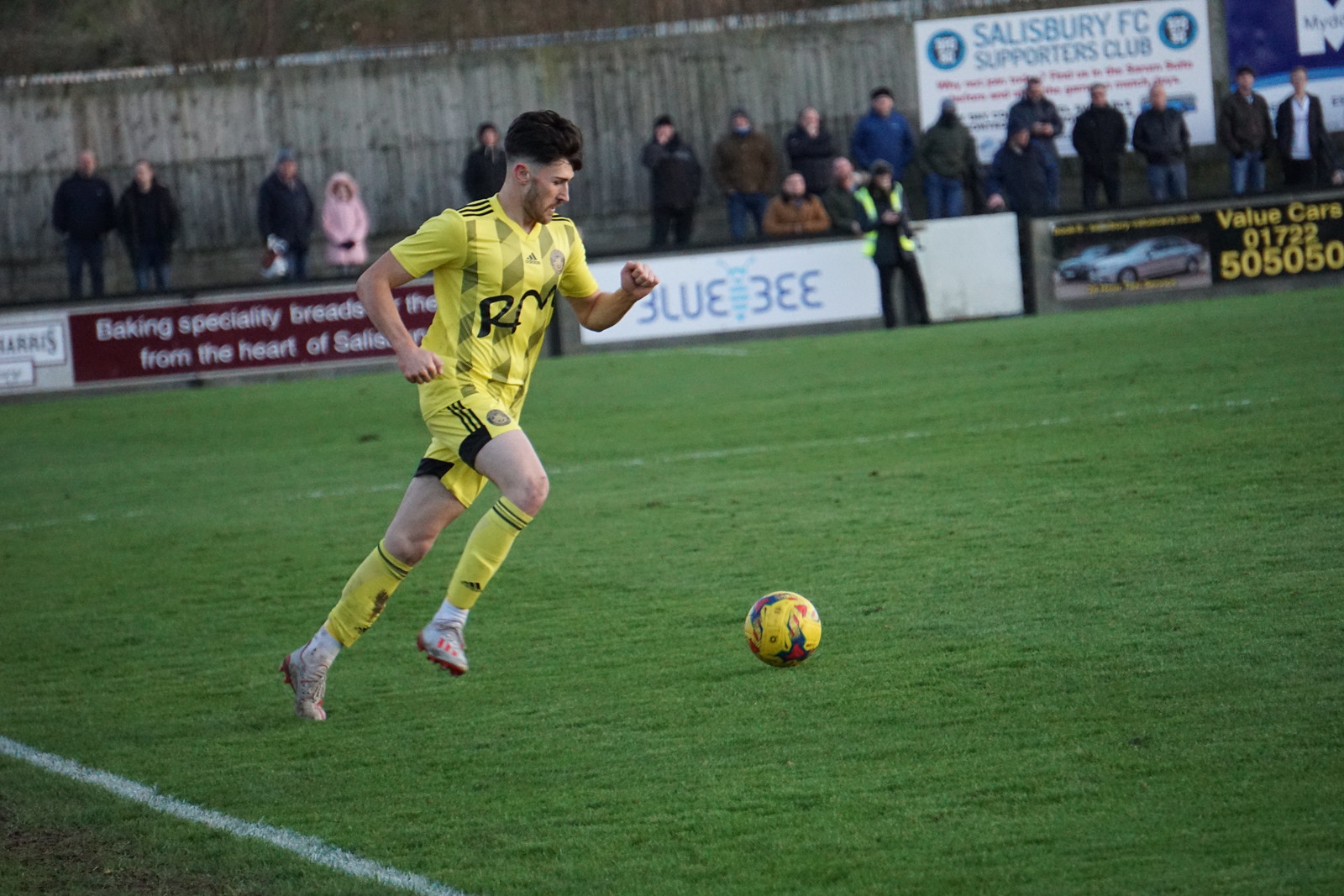In this highly detailed and sharp photograph, a soccer player is captured in the foreground, poised to kick a yellow ball. The player is centrally positioned on a vibrant green pitch, donned in a green and yellow uniform with "R.M." in modern font on the jersey, complemented by yellow socks. The background, slightly out of focus, shows spectators in warm apparel, including coats, caps, and even a parka with a hood, indicating chilly conditions. Additionally, there's an official in a colored vest, similarly dressed in warm clothing with a cap and heavy coat. The stadium's boundary is lined with advertisements for brands such as Blue Bee, Value Cars, and specialty baking breads, adding to the vividness of the scene. On one side, there is mention of "Salisbury Football Club" and "Supporters Club." This clear and sharp photograph beautifully captures a moment of anticipation in the game with a well-defined player against the lively backdrop of engaged fans and colorful ads.